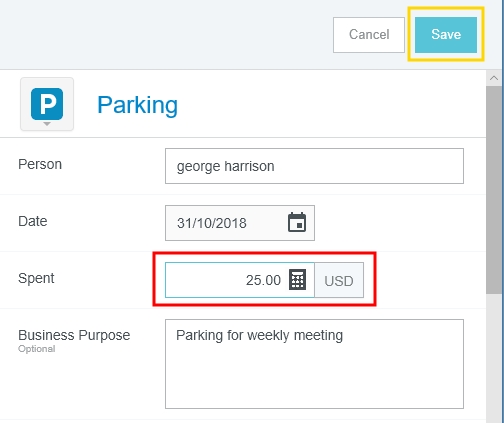This screenshot detailing a parking record is square-shaped with a white background. A prominent wide gray banner spans horizontally across the top, and on the right side of this banner are buttons labeled "Cancel" and "Save," with the "Save" button distinguished by a yellow outline. Central to the page is a parking icon, represented by a blue square featuring a gray "P" in the center. Adjacent to the icon, the word "Parking" is displayed. Below this, a thin horizontal gray line separates the section detailing specific information. 

This includes a field labeled "Person" with the name "George Harrison" filled in. The date indicated is "31-10-2018." Directly below, a box labeled "Spent" is outlined in red, showing an expenditure of "$25." An adjacent field, titled "Business Purpose" and marked as optional, contains the note "Parking for weekly meeting."